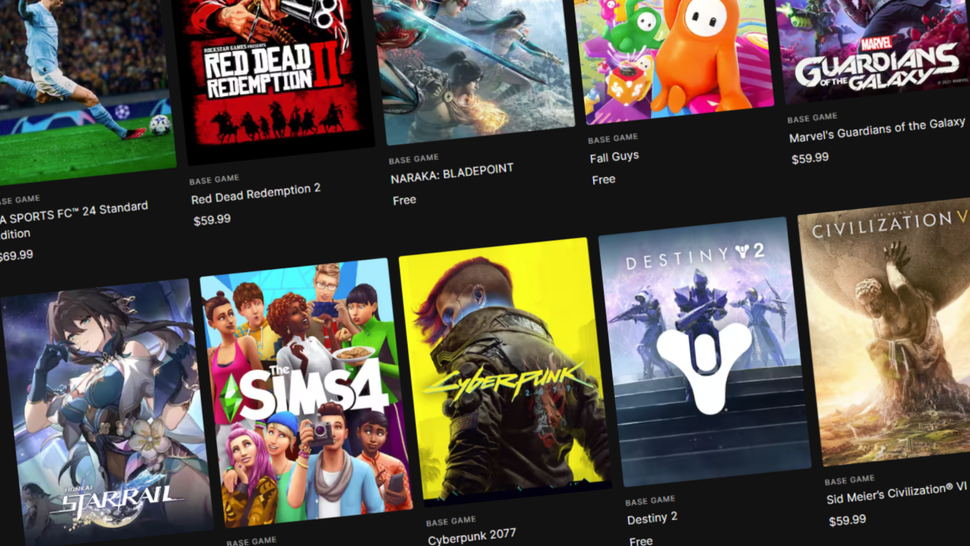A screenshot captured from a video game company's website showcases a selection of video games available for digital purchase. The image is taken at a slight angle, transitioning diagonally from the upper right to the bottom left corner. It displays a variety of games, each accompanied by a visual thumbnail and pricing information. 

Prominently featured at the top left is "Sports FC 24 Standard," highlighted by an image of a player kicking a soccer ball, priced at $69.99. Next, "Red Dead Redemption 2" is presented with a vibrant red theme, priced at $59.99. Following that is "Naraka: Bladepoint," listed as free, and "Fall Guys," also available for free.

Below these titles, "Marvel's Guardians of the Galaxy" appears, priced at $59.99, while an anime-styled game, possibly named "Starvale," is displayed next to "The Sims 4." Further down, "Cyberpunk 2077" and "Destiny 2" (free) are listed. Lastly, the strategy game "Sid Meier's Civilization 6" is shown, priced at $59.99, with the thumbnail partially obscured, revealing only the letter "V."

This screenshot, clearly from an online video game store, highlights a mix of free and premium games, with several titles priced primarily at $59.99 or $69.99.